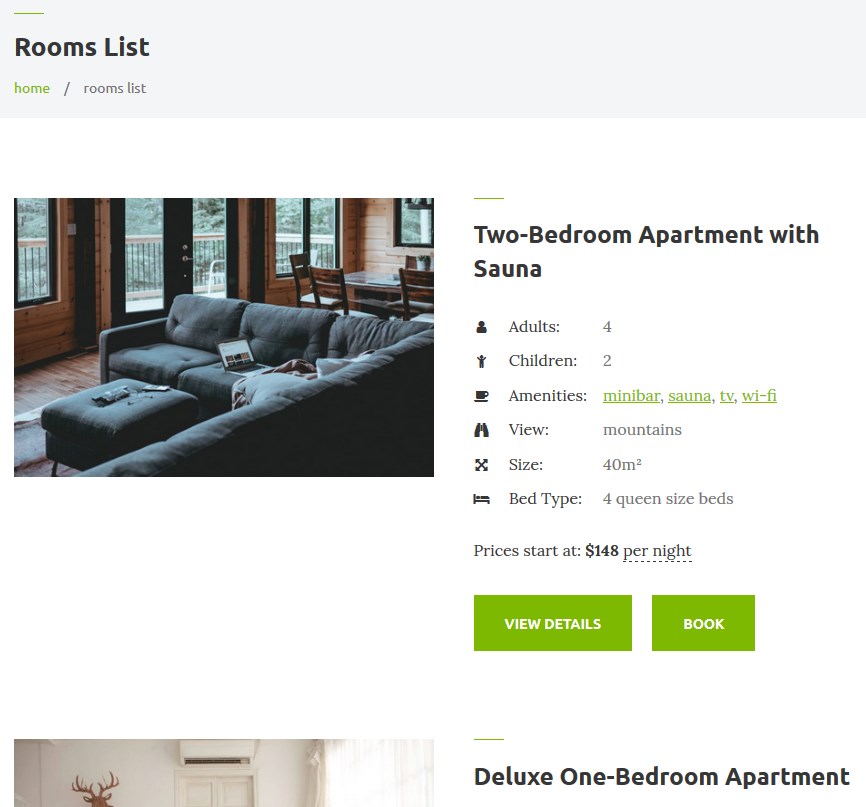Image Description: 

The image is a screen capture from an online application with a white background. In the upper left corner of the screen, the text "Rooms List" is written in black. Directly below that, there is a breadcrumb trail that reads "Home / Rooms List." 

Underneath this, there are two images displayed. 

The first image, located on the left side, depicts the interior of a living room. The room features a dark gray sectional couch with a matching Ottoman placed in the center. The walls are made of wood, creating a warm and inviting atmosphere. Large glass doors with black door frames provide a view of the outdoor patio railing and the surrounding trees.

To the right of this image, black text reads "Two Bedroom Apartment with Sauna." Below this heading, several details are listed:
- Adults: 4
- Children: 2
- Amenities: Minibar, Sauna, TV, and Wi-Fi (written in green text).